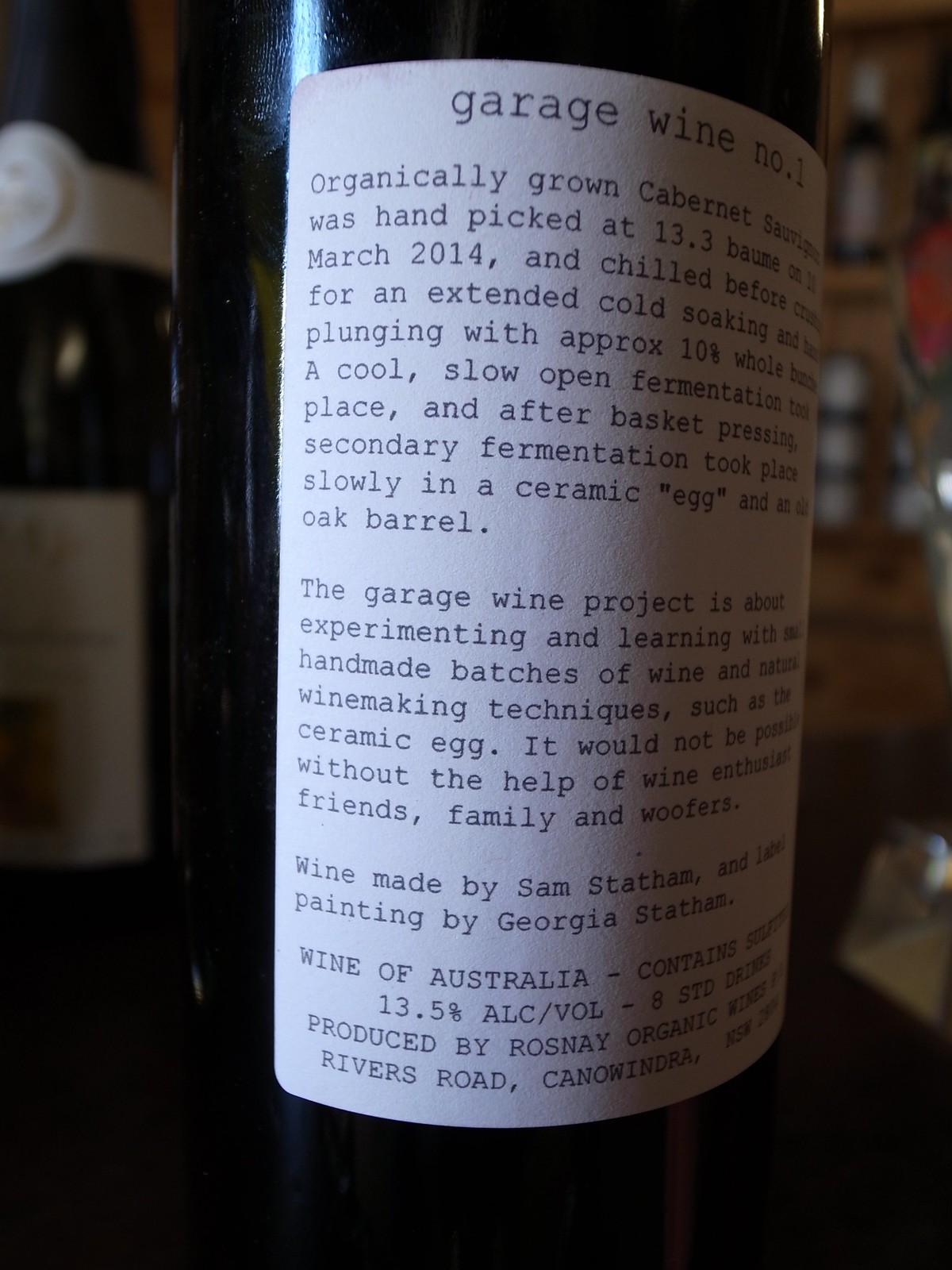This is a close-up photo of a dark wine bottle with a predominantly white label, set against a backdrop that suggests a wine store. The bottle, labeled "Garage Wine No. 1," stands out with a homemade aesthetic, featuring text reminiscent of a typewriter. The label specifies that the wine is an organically grown Cabernet, with hand-picked grapes harvested in March 2014. The camerawork only partially captures the text as the right side is obscured by shadows and the bottle's curvature, but it highlights that the wine underwent a unique fermentation process, including extended cold soaking, plunging, and slow fermentation in a ceramic quill egg and oak barrels. The alcohol content is 13.5%, and it is produced by Rossini Organic Vineyards, located on Rivers Road, Australia. To the left of the bottle, another wine bottle is faintly visible, and the background includes what appears to be more wine bottles and a large case wrapped in white.